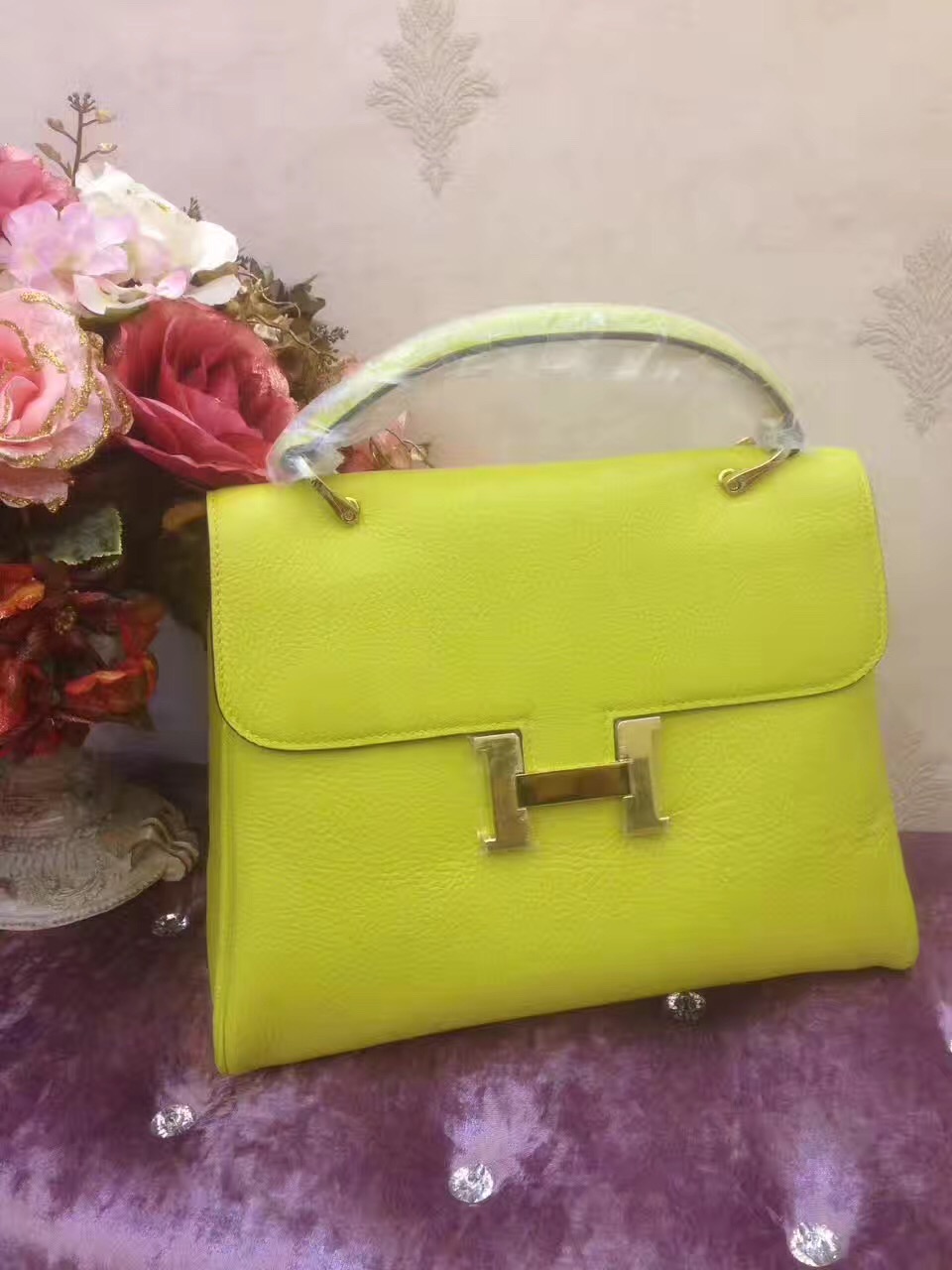This still life image features a striking yellow handbag adorned with a gold buckle on its front, reminiscent of an "H." The purse, complete with a carrying handle still covered in protective plastic, is set on a distinctive purple cushion, which appears to be upholstered with diamond-studded details. To the left of the purse, a beautiful bouquet of flowers, including pink, white, and burgundy blooms, sits atop an ornate stone base with gold decorations. The scene is set against a white wall featuring subtle leaf patterns, adding an elegant backdrop to the composition.